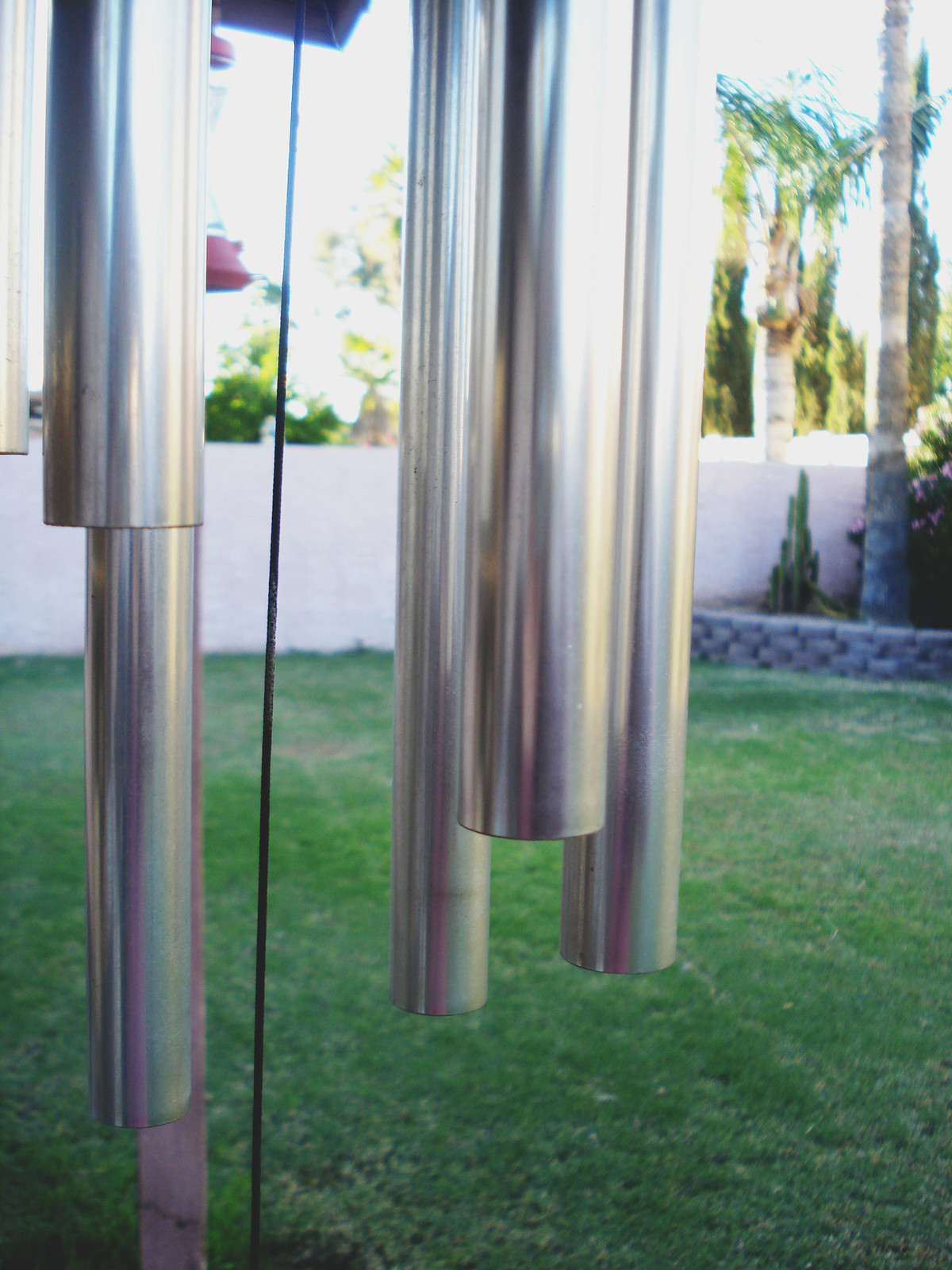A close-up colour photograph captures contemporary stainless steel wind chimes featuring long cylindrical poles. The wind chimes, appearing quite long and almost reaching the ground, dominate the foreground. In the background, a lush yet slightly patchy green lawn stretches across the scene, with some brown patches hinting at soil. A white painted brick wall, likely marking the garden's boundary, runs horizontally through the centre of the image. To the back right, an orderly raised flower bed made of alternating dark grey bricks without mortar houses a variety of plants. A tall palm tree trunk, with its characteristic horizontal stripes of light and dark brown, emerges from this flower bed, extending upwards and out of the frame. Adjacent to the wind chimes, a clear hummingbird feeder with a red top and bottom dangles from a long pole. The garden showcases meticulously cared-for landscaping, with evergreens and flowering bushes adding to its charm. The bright, sunny sky in the background creates a slight overexposure, blurring the distant view but highlighting the serene outdoor setting.